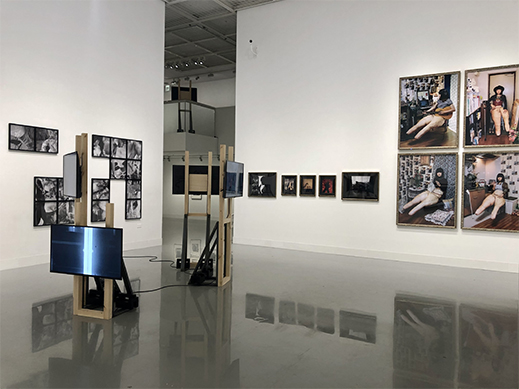This full-color photograph captures an indoor art gallery, illuminated by artificial light. The square image features highly polished floors that reflect the vivid artworks displayed on the white walls. The gallery's ceiling showcases a distinct grid pattern. 

On the far right wall, there are four large paintings depicting the same woman in various poses. This woman, with long black hair, appears to be a left-handed guitarist, strumming her instrument while wearing a shirt but no pants. 

In the center of the gallery, smaller paintings are arranged vertically. The left wall holds an array of additional works, including smaller black and white photographs and colored images. In the lower left-hand corner, a video screen is visible, next to a wooden structure supporting two monitors. Another video installation features a stark bluish-white neon line down its center. Overall, the gallery presents a cohesive and immersive visual experience.